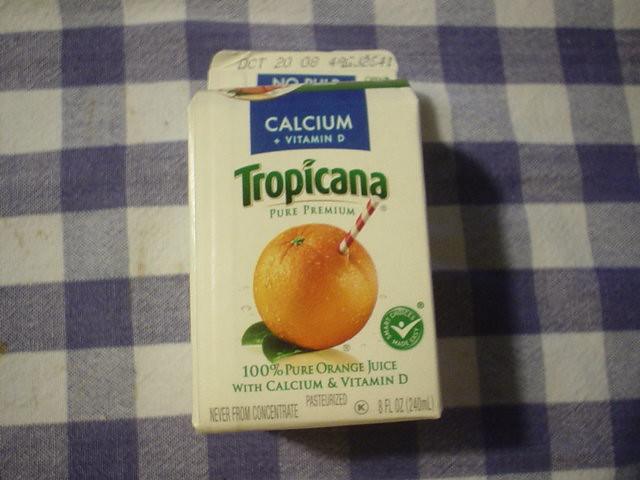This photograph captures a slightly worn and tattered small 8-ounce carton of Tropicana orange juice, viewed from above, placed on a dark navy blue and white buffalo check fabric. The carton, which is ivory in color with prominent green text, is positioned slightly on the bias towards the upper left corner. The top of the carton is crumpled, displaying an expiration date of "OCT 20 08" along with some other digits. 

At the very top, in a blue rectangle, there is text reading "NO PULP" followed by "CALCIUM" and "VITAMIN D" in white capital letters. The front features the word "Tropicana" in an arched shape in green letters, followed by "Pure Premium." The central image on the carton is of an orange with two green leaves at the bottom and a red and white striped straw inserted into it. Below this image, the text reads "100% Pure Orange Juice with CALCIUM and VITAMIN D, Pasteurized." Further down is a green circle with a white checkmark, indicating some form of quality or approval.

On the lower right-hand side, it states "8 FL OZ (240 ML)" and on the left-hand side, "NEVER FROM CONCENTRATE" is written in green. The carton is lying flat on the checkered cloth, casting a shadow across the fabric.